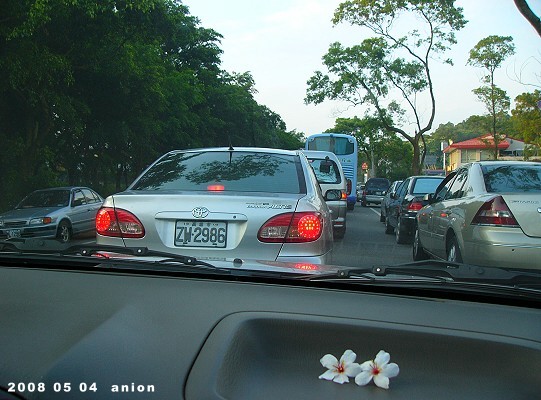In this rectangular photograph, we glimpse a scene from the passenger seat of a car, peering out through an unobstructed windshield. The sleek, black dashboard is accentuated by two small white flowers resting on its surface, located in the lower right corner of the image. Ahead, a bustling stretch of road features two lanes filled with various vehicles, including sedans and larger automobiles. In the distance, a distinctive blue bus is visible. The scenery is set against a backdrop of a light blue sky, adorned with scattered white clouds. The date is marked in the lower left corner of the photograph, reading "2008-05-04," accompanied by the text "ANEON" in small print.